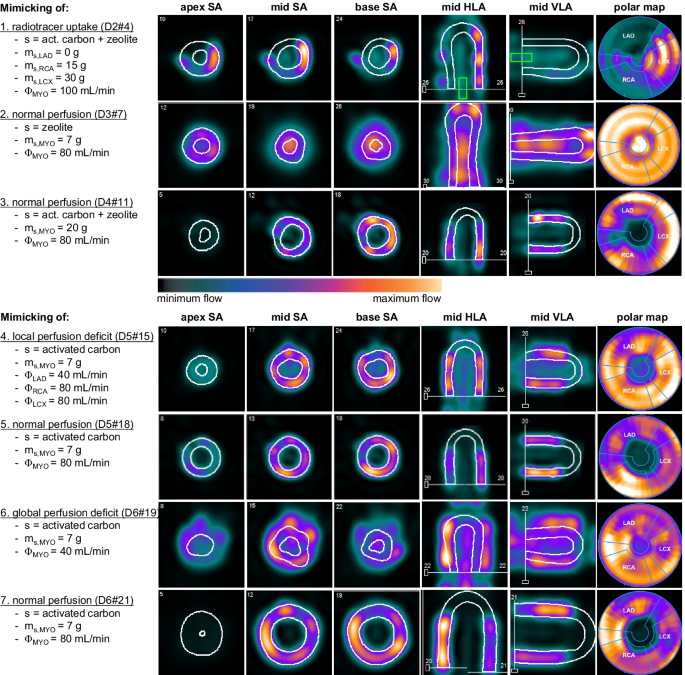This image presents a detailed scientific chart with a series of vivid, colorful diagrams arranged in columns and rows. Each column is marked with titles indicating specific anatomical perspectives, such as Apex SA, Mid SA, Base SA, Mid HLA, Mid VLA, and Polar Map. The sections are divided into equal square segments, all featuring a black background and containing dynamic color gradients representing various data points. These gradients display progression from blue and green (indicating minimum flow) through purple, pink, and red, to orange and yellow (indicating maximum flow).

On the left side of the chart, there are numerous mathematical equations and notations detailing the information represented in the diagrams. These mathematical annotations outline radio tracer uptake, including details of normal perfusion and perfusion deficits across various ranges (D3-7, D4-11, D5-15, D5-18, D6-19, and D6-21). The notations align with a numerical order from 1 to 7, each corresponding to one of the colorful diagrams in the chart.

Starting from the rightmost Polar Map, each diagram begins with a circular design that gradually expands before transforming into more complex shapes, culminating in the characteristic 'horseshoe' magnet shape. The VLA to Polar Map transition shows the progression into a full circle with a smaller, color-void interior circle. This detailed layout, replete with heat signal visualizations, captures the variance in cooler to hotter regions as indicated by the blue-to-yellow color spectrum.